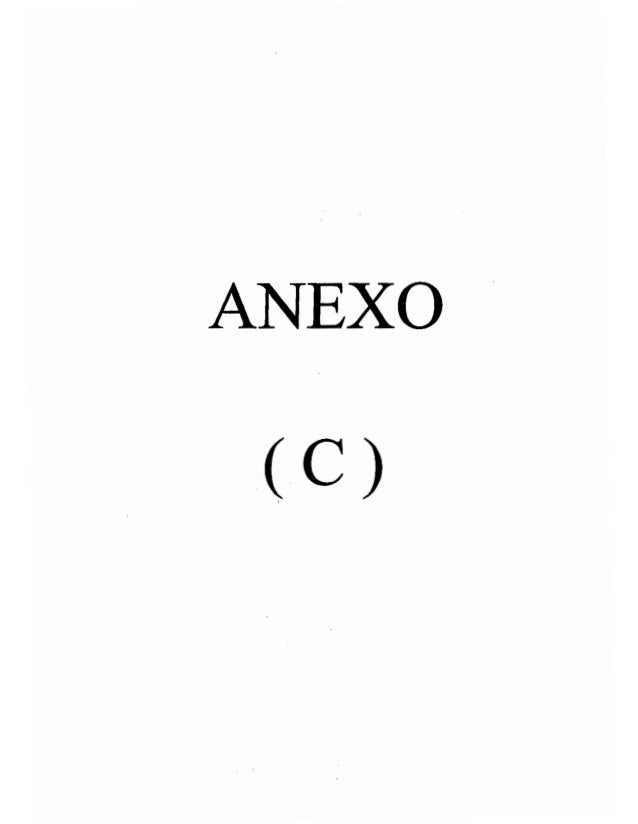The image features a very simplistic and clean design with the black capital letters "A-N-E-X-O" typed in what appears to be a Roman Arial font. The letters, slightly resembling typewriter text with a blotchiness suggesting faded ink, are centrally positioned towards the upper part of the image. Below the letters, there is a significant gap followed by a capital "C" enclosed in parentheses, commonly indicating a copyright symbol. The background is entirely white with no other elements present, lending to the stark and minimalistic feel of the image.